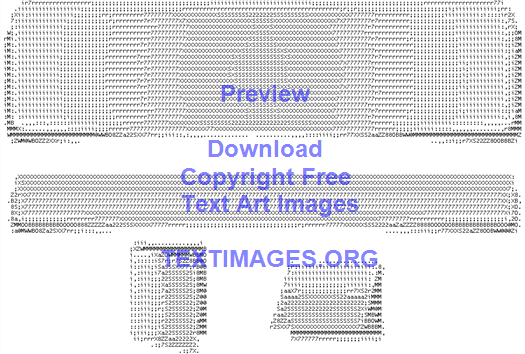The image is a computer-generated artwork composed of various symbols, including numbers, dots, letters, and question marks. The backdrop features a white mesh or nylon netting pattern. Centrally positioned in blue text, it reads "Preview, Download, Copyright-Free Text Art Images," followed by "textimages.org." At the top is a large rectangular shape resembling a band-aid, which casts a shadow due to bold symbols. Below it is a long rectangular shape with a shadow effect. Further down are two smaller shapes: one appears like a folded piece of paper, similar to a greeting card, and the other like an irregularly shaped book. The colors in the image are limited to black, white, gray, and blue.